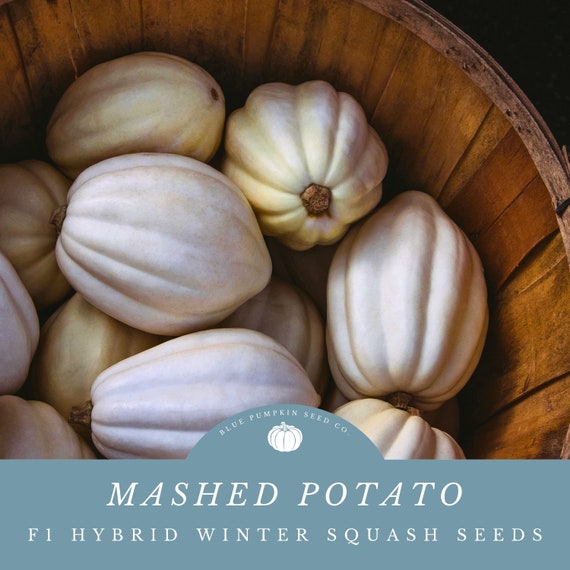The flyer features a prominently displayed wooden basket brimming with small, off-white squash that resemble a cross between a papaya and traditional squash, with a more rounded shape. These neatly stacked squashes are presented in a cozy, rustic fashion. Dominating the bottom portion of the flyer is a light blue banner with bold white text that reads "Mashed Potato F1 Hybrid Winter Squash Seeds." Above this banner, taking up the upper part of the flyer, is the logo of "Blue Pumpkin Seed Co.," featuring a white pumpkin illustration. The overall background of the flyer includes subtle hints of a black backdrop, heightening the focus on the wooden basket and its unique contents.